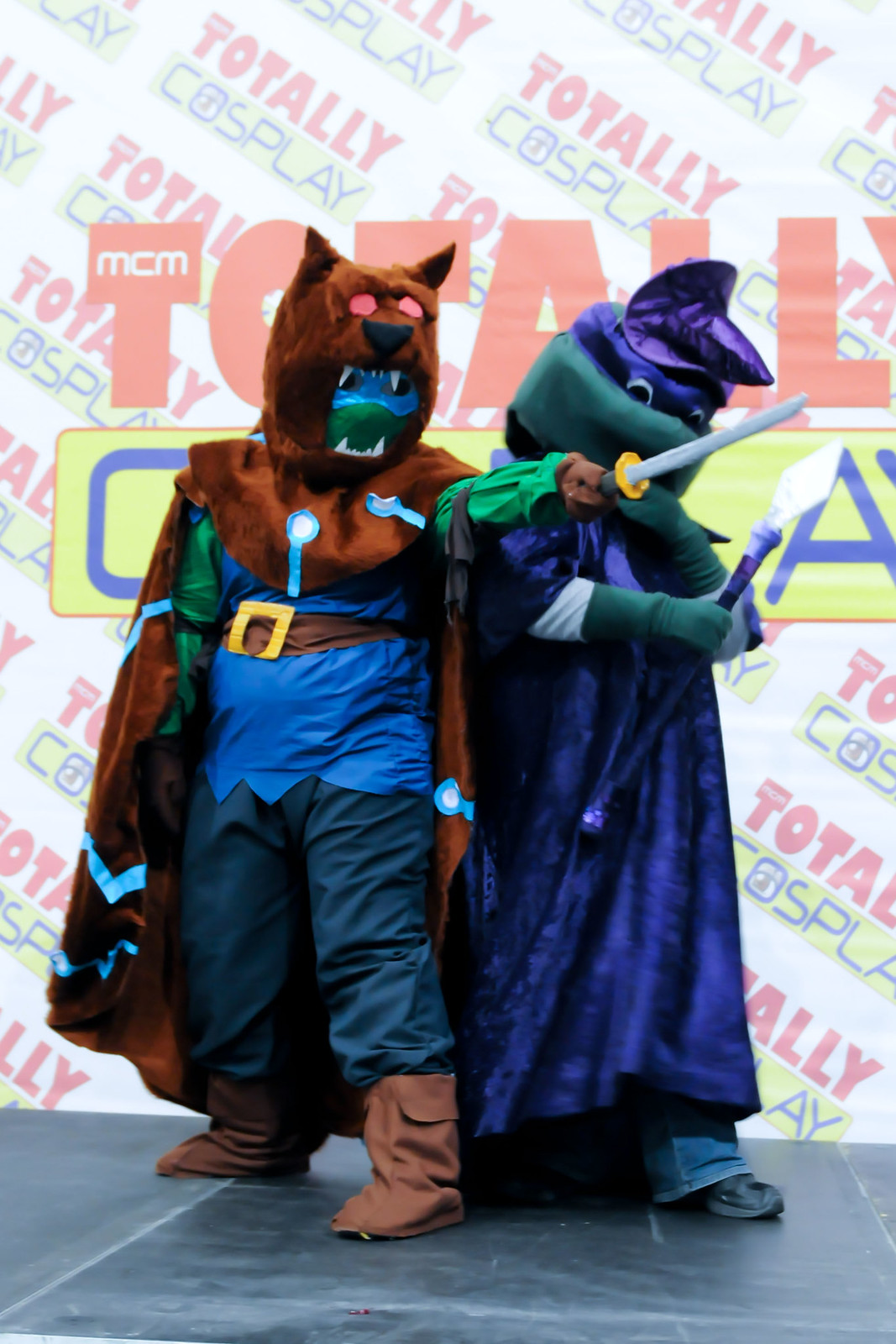The image showcases two cosplayers posing in front of a large, vibrant sign that reads "TOTALLY COSPLAY," with "TOTALLY" in bold red letters and "COSPLAY" in blue letters against a yellow rectangle. The cosplayers stand on a gray platform, possibly a stage, under what appears to be natural lighting.

The cosplayer on the left is dressed in a unique ensemble that blends elements of a bear and a swashbuckler. They wear a large bear mask over a green interior headpiece with a blue mask, paired with a blue shirt, blue pants, a cape, and a yellow-buckled belt. Their outfit is complemented by gray or brown boots. They appear to be holding a sword, accentuating their adventurous look.

On the right, the second cosplayer embodies a strikingly unconventional character that suggests a wizardly Teenage Mutant Ninja Turtle. They sport a large green head with a purple eye mask, a purple robe, and a purple hat that is slightly askew. They wield what could be a magic staff or spear, further enriching their wizard-like appearance. This cosplayer also wears green gloves, completing the head-to-toe transformation.

Overall, the juxtaposition of these imaginative costumes against the "TOTALLY COSPLAY" backdrop vividly captures the playful and creative essence of cosplay.